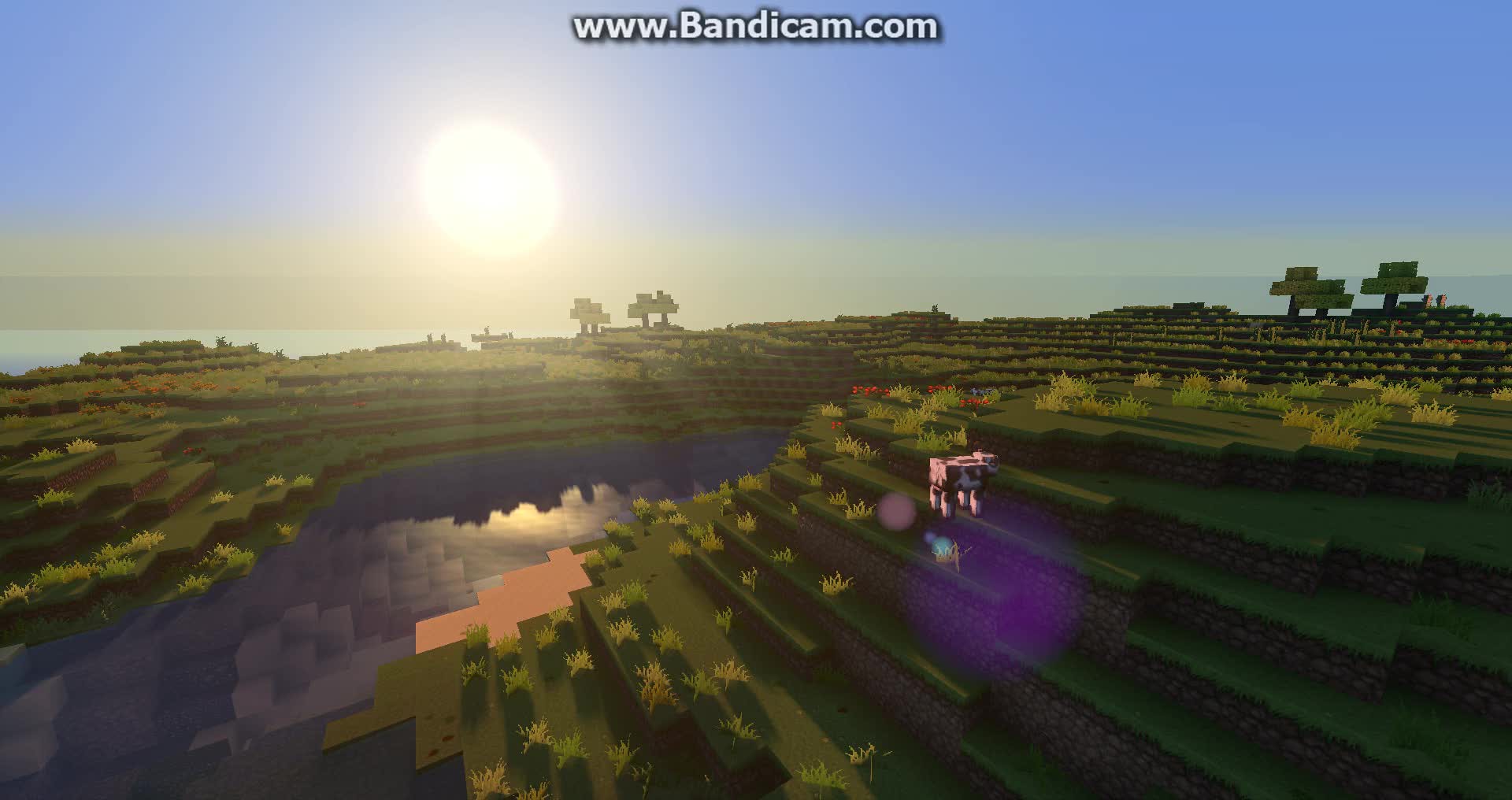This screen capture from a computer game features a pixelated, panoramic landscape. Prominently, "www.bandicam.com" is displayed in white text at the top center. The scene depicts a vibrant and verdant environment with a distinctly blocky aesthetic, reminiscent of a Lego-like or cartoon style. In the distance, a bright yellow sun illuminates the sky, which is streaked with horizontal lines, possibly indicating a haze or clouds. The horizon showcases blocky hills adorned with chunky trees. 

The foreground highlights a terraced slope constructed from stone walls and layered steps of greenery. Textures range from short vegetation to larger bushes ascending the terraces. A blocky body of water and a patch of similarly styled beach further add to the scenery. A distinct feature is a square cow with bowling pin-like legs standing on the green slope, emphasizing the whimsical, pixelated design of the terrain. This intricate depiction underscores the game's stylistic choice of a blocky, computer-generated world filled with life and features.